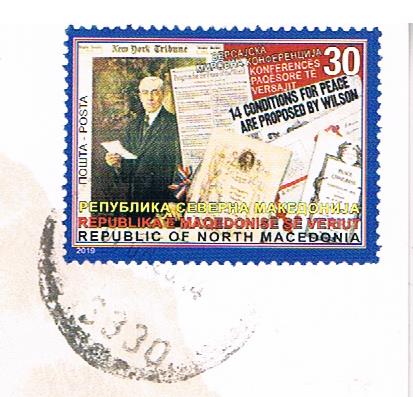The image is a detailed close-up of a color postage stamp from the Republic of North Macedonia, affixed to a letter and marked with a postmark. The stamp has a dark blue border and features a prominent portrait of an older man, presumably Woodrow Wilson, wearing glasses and a black suit with a white shirt and tie, holding a white document. The left side of the stamp showcases the words "New York Tribune" and includes a portion of a historical image from the newspaper. The background incorporates various articles and images related to Wilson, with a specific headline reading "14 conditions for peace are proposed by Wilson." Written in multiple languages, including Russian and Macedonian, the stamp also prominently displays "Republic of North Macedonia" at the bottom. The top right corner of the stamp features a red background with the number "30" in white text, and the design uses a color palette of red, yellow, black, white, and blue. The overall style is photographic representationalism, and the stamp's indicia partially obscures the lower left corner.